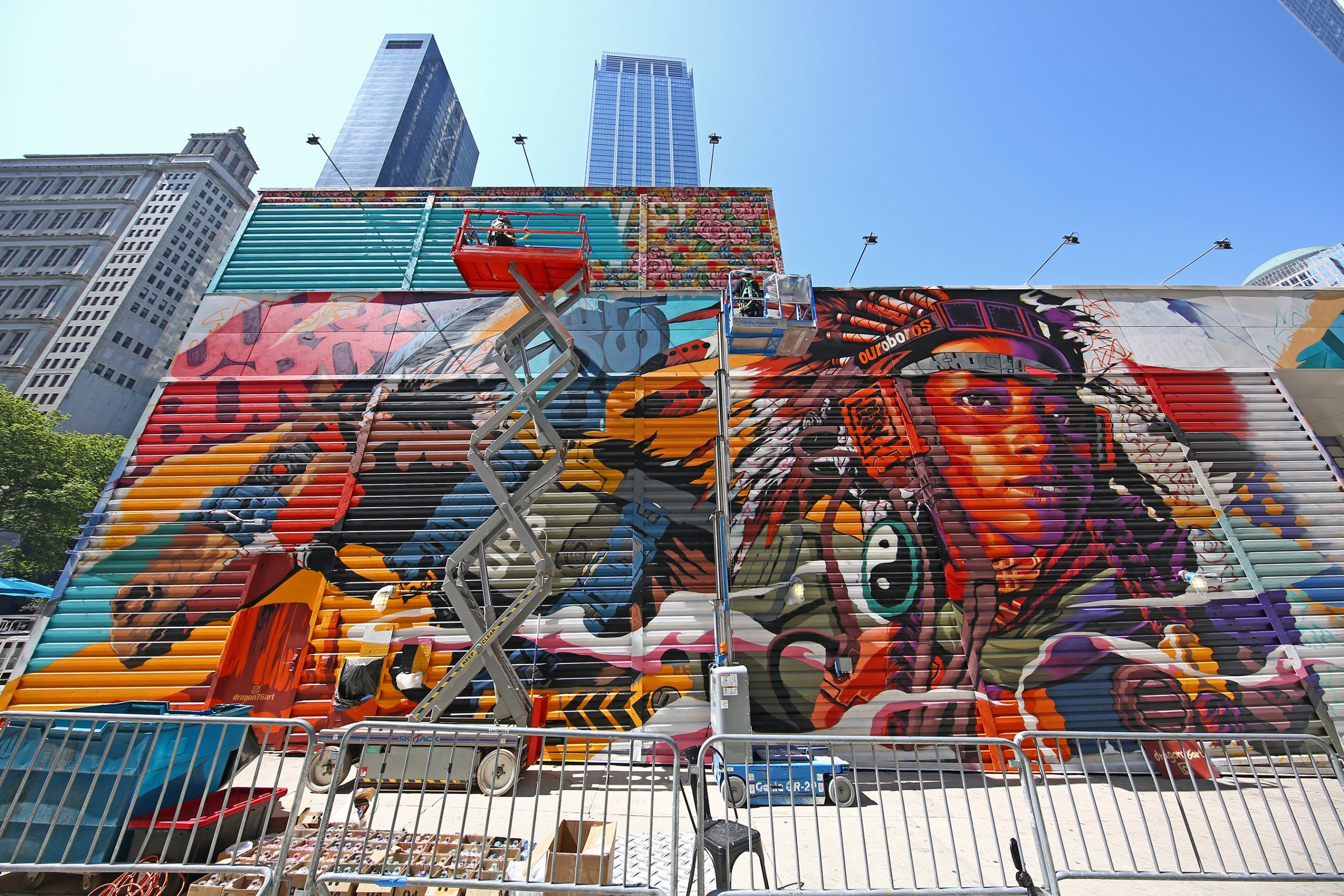The photograph, taken during the daytime in an urban area, captures a vibrant mural painted on the side of a building, likely in New York. The mural is a striking and colorful depiction of an indigenous woman turning to the right, with reddish-brown skin and a contemplative expression directed downward at the viewer. She wears a headdress adorned with beads and feathers flowing back, and a yin-yang emblem is prominently featured on the left side of her face, enhancing the blend of traditional and modern artistic elements. The mural, currently in progress, features a large gray crane supporting the artist, who is actively painting the piece—a style known for its photographic representationalism and realism by street artist Dragon76. In the background, several towering skyscrapers dominate the skyline, while the scene at street level includes a silver fence, a red platform, and a few trees partially framing the image. The blue sky overhead adds a further sense of depth to this urban landscape.